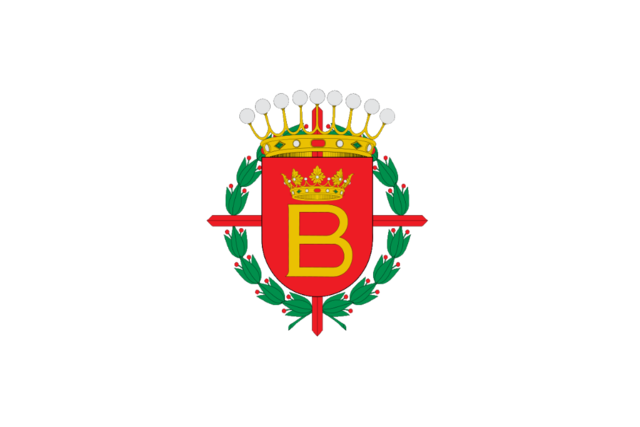This detailed logo features a central red shield adorned with a gold letter 'B'. Atop the 'B' rests a golden crown, embellished with green, white, and red jewels as well as large white beads lining its top. Above this crown, an additional, larger crown sits, enhancing the emblem's regal appearance. This entire ensemble is set against a red cross, further highlighting the shield. Encircling these central elements is a lush green wreath interspersed with red berries. The background of the image is predominantly white, making the intricate details of the logo stand out prominently.